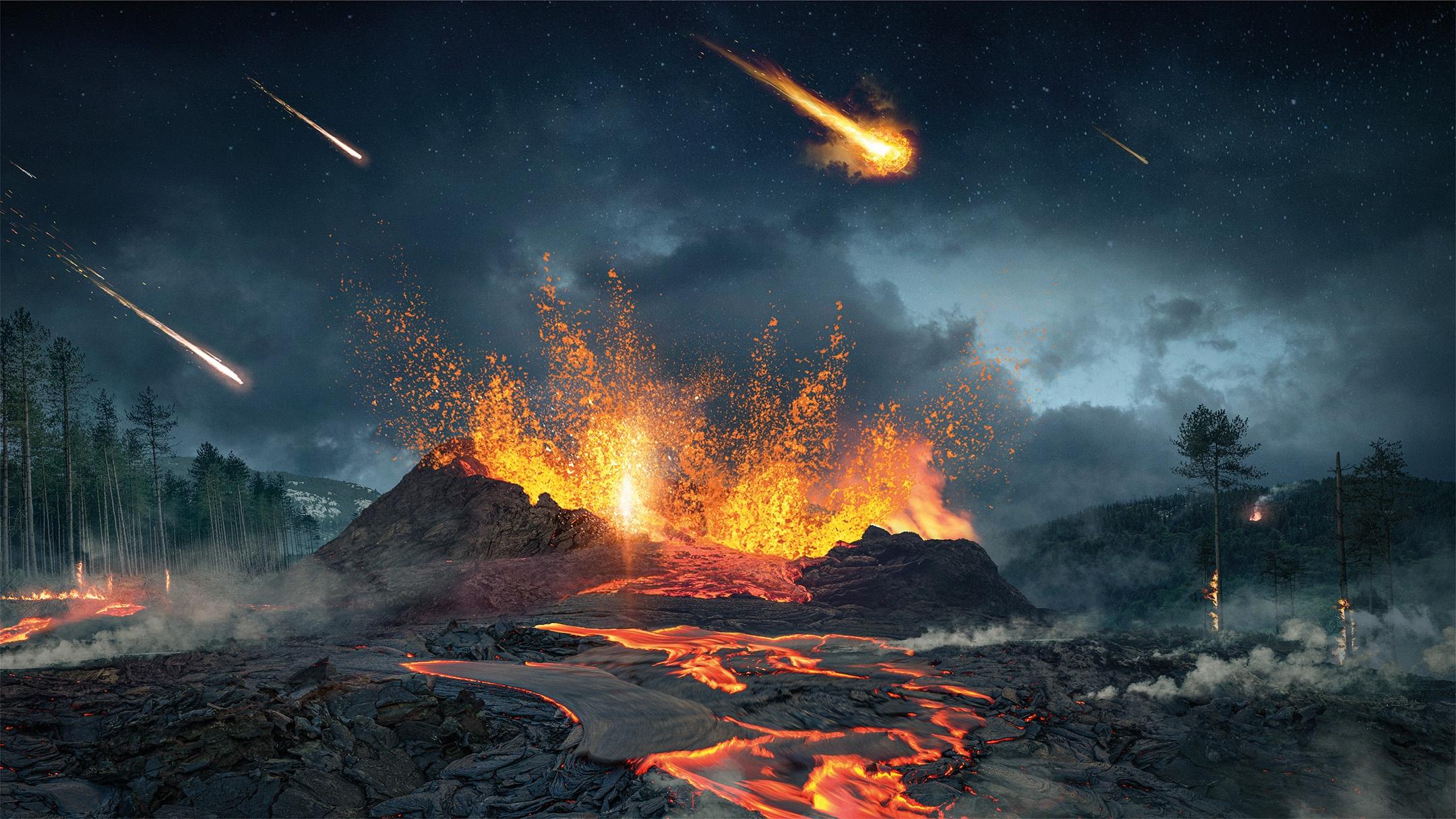This image, likely a combination of CGI and digital enhancements, depicts a highly detailed and fantastical volcanic eruption scene. In the center foreground, a short volcano is actively erupting, spewing a vivid mix of red-hot, molten lava, and partially cooled magma that flows dynamically towards the viewer. The ground around the volcano is scorched and blackened, with several areas still smoldering and smoking. Surrounding the volcanic crater, tall trees flank both sides, many appearing bare at the base with foliage only at the top, while others are already succumbing to the advancing flames. 

In the backdrop, the sky transitions from a dark, smoky expanse to patches of star-studded night sky, punctuated by clouds illuminated by the fiery landscape below. Fiery comets or meteors streak dramatically across the scene, the largest one blazing prominently in the sky and trailing smoke. In the distance, a snow-capped mountain and a fire-engulfed hill add to the apocalyptic ambiance. The overall effect is a luminous, dynamic tableau of natural disaster and surreal celestial phenomena.